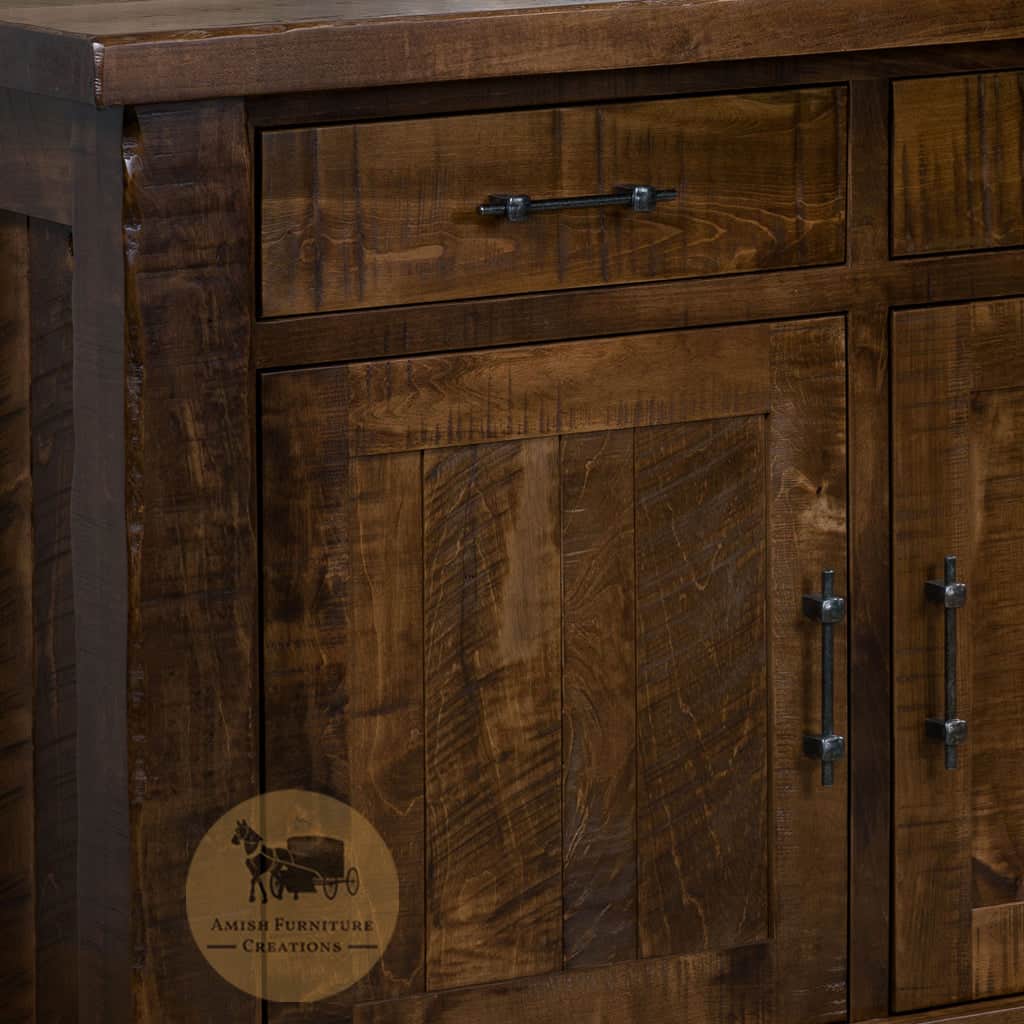The image showcases a dark brown, polished hutch-style piece of furniture, likely suitable for a kitchen. The wood has a refined, aged look with detailed craftsmanship, exhibiting both darker and lighter shades of brown, and features a wooden-like design. The furniture includes two top drawers and two bottom cupboards with matching black, iron-like handles. The drawer handles are thin metal bars placed horizontally, while the cupboard handles are positioned vertically, each with a central line and knobs on either end.

In the bottom section of the furniture, there is a tan, semi-transparent circle containing an artwork of a horse pulling a carriage, rendered in black. Below this illustration, it reads, "Amos Furniture Creations," celebrating the artisanal quality of the piece.